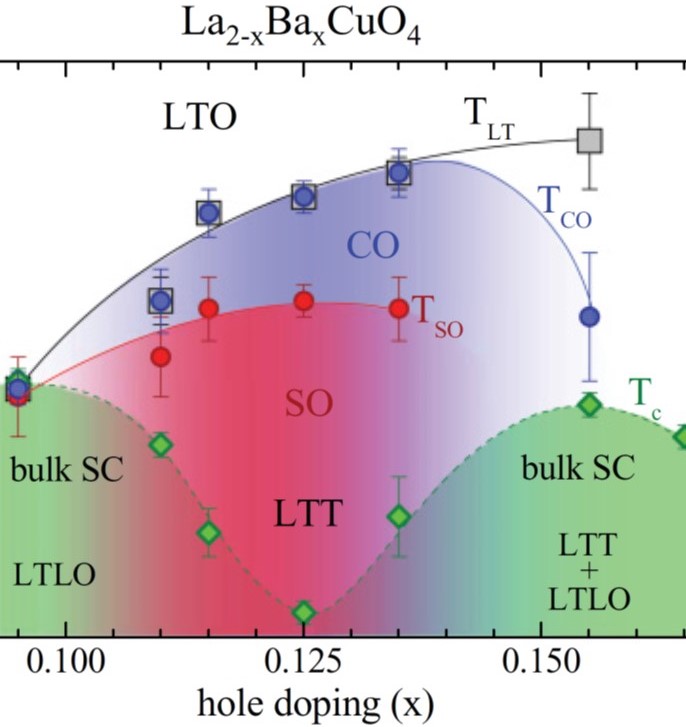The image is a detailed scientific chart set against a white background. It features two horizontal black lines, one at the top and one at the bottom, resembling ruler markings. At the top, in black print, it reads "LA2-XBAXCU04" with an underscored line below it. Below the top line, the labels "LTO" and "TLT" are present. The chart is marked by numbers at the bottom: 0.100, 0.125, and 0.150, with indicators of whole doping denoted by "X" in parentheses. The graph features several curved lines: one is a waved line with green dots descending from left to right, while others are curved lines with blue dots arcing upwards. The graph also includes a color-coded section: green in the bottom left and right labeled "Bulk SC LTLO" and "Bulk SC LTT + LTLO" respectively, and a red section in the middle annotated with "LTT and SO." The upper area of the graph is shaded purple. The data points on the lines are symbolized by blue diamond shapes inside gray squares outlined in black.